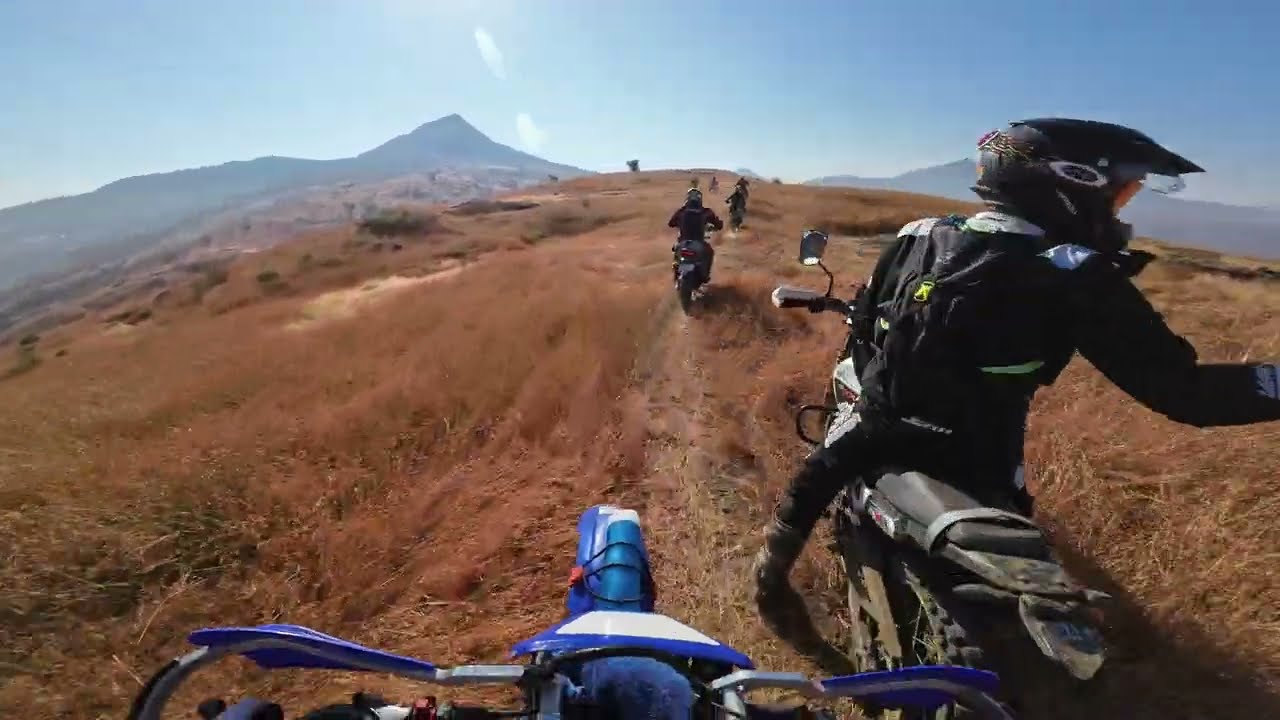The photograph depicts a sunny day with a clear, blue sky and a range of mountains in the background. The scene is viewed from the perspective of someone on a blue motorcycle, evident from the handlebars visible in the lower middle of the image. The dirt path winds through a grassy hillside covered in brown, dry brush. In front of the blue motorcycle, to the right, is another motorcyclist dressed entirely in black, including a black helmet and a small backpack. This rider seems to be looking over their right shoulder. Farther along the trail, several other motorcyclists are visible, making their way towards the distant hills. The overall composition captures the dynamic movement and camaraderie of a group of motorcyclists navigating a rugged, scenic route.